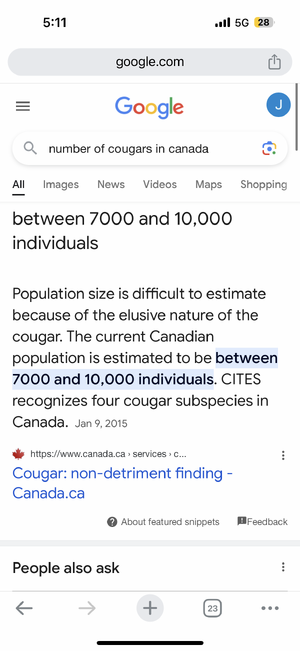This screenshot captures a mobile view of a Google search page, and it provides various details from the screen's layout. At the top of the screen, in bold black letters, "Google" is displayed. The time is shown as 5:11, towards the far right of the status bar, signal bars can be seen alongside a "5G" indicator and a battery icon which is depicted as yellow, indicating a 28% charge remaining. 

A gray oval with "Google.com" text is visible below the status bar. The iconic Google logo, composed of multicolored letters, is centered prominently at the top of the search page. To the far right is a blue circle containing a white "J", serving as the user's avatar.

The search query, "number of cougars in Canada," is displayed, with the search results page set to the "All" tab. The main search result summarized states: "Between 7,000 and 10,000 individuals." This number is highlighted in blue text. It is noted that "The population size is difficult to estimate because of the elusive nature of the cougar." The statement is further detailed as: "The current Canadian population is estimated to be between 7,000 and 10,000 individuals."

Below this, the text continues with, "Sites recognize four cougar subspecies in Canada," featuring a small red Canadian maple leaf beside it. The source link is abbreviated as, "https://www.canada.ca...", which leads to the titled page "Cougar Non-detriment Finding Canada.ca." 

Additionally, the "People also ask" section is briefly visible but mostly cut off.